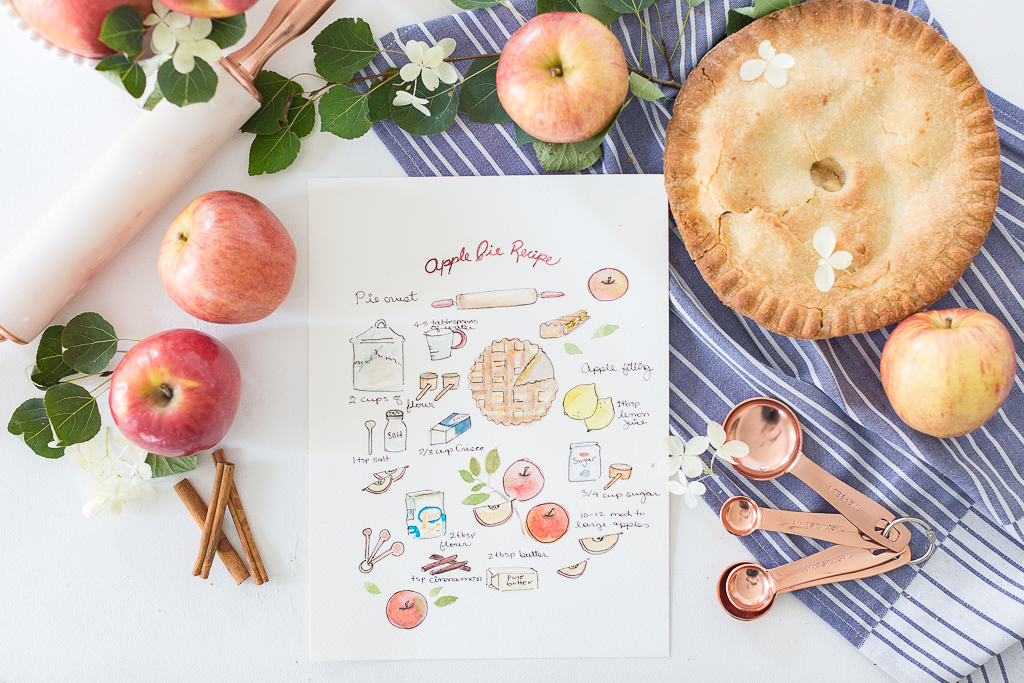The photograph captures a top-down view of a white table adorned with a blue and white striped tablecloth or dish towel on the right. At the heart of the composition is a baked apple pie, adorned with a few small white flowers and a hole in the center revealing the apples inside. Scattered around the table are four apples, cinnamon sticks, copper measuring spoons, and a white rolling pin with copper handles. Adding to the scene's charm, there are apple blossoms and greenery interspersed throughout. Positioned centrally is a white sheet of paper titled "Apple Pie Recipe," which features a whimsical, illustrated guide to making the pie, complete with labels and colored drawings of ingredients like apples, pie crust, and utensils. The overall aesthetic is simple and inviting, reminiscent of a Nancy Meyers film.